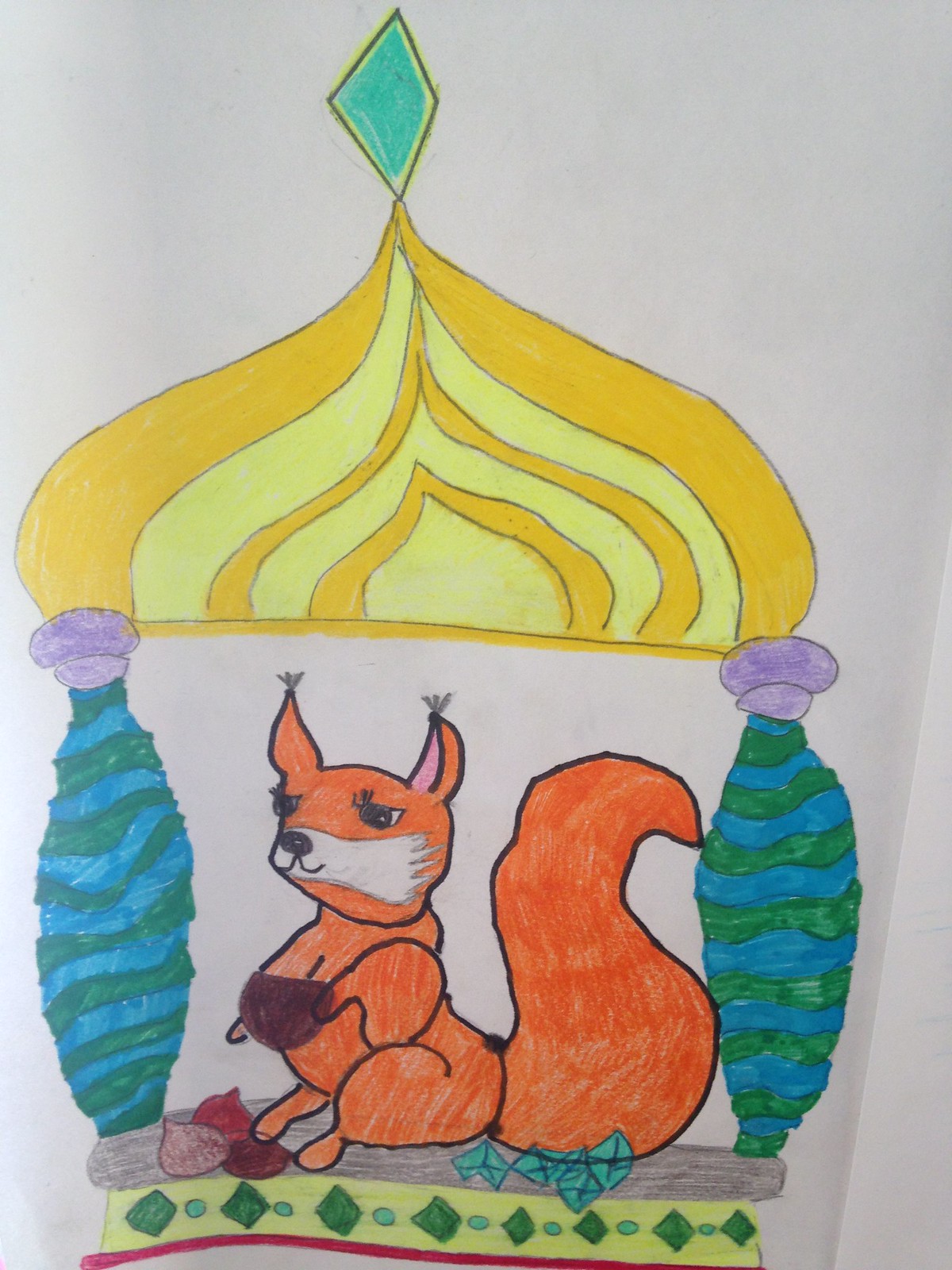This is an intricate child's drawing rendered on off-white paper using vibrant markers. Central to the composition is an orange fox squirrel, distinguished by its white snout and cheeks. The squirrel's alert expression is accentuated by its pointy ears, each adorned with a tuft at the tip. Flanking the squirrel are two swirled columns in green and blue, capped with ornate purple balusters. Above the scene, an onion-shaped dome in yellow and gold hovers like a fantastical roof, crowned with a blue diamond at its apex. The squirrel clutches a small, dark brown acorn, with several more scattered on the ground before him. Additionally, numerous tiny blue diamonds adorn the area around the base of the squirrel's bushy tail, adding a touch of whimsy to the detailed scene.